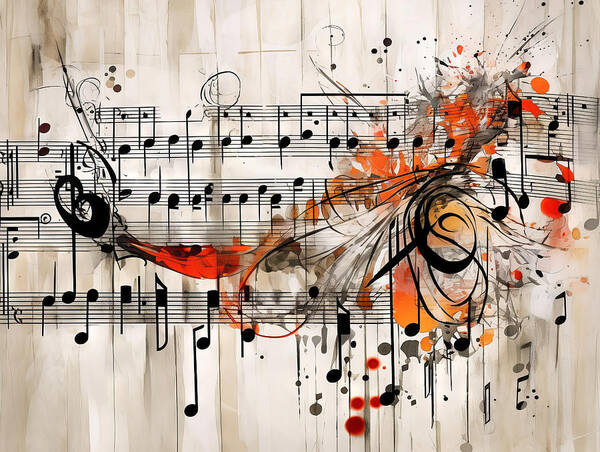The image is a horizontal rectangular piece of abstract art centered around a sheet of sheet music with an off-white background. The music notes are predominantly black, organized into two stanzas with rich, intricate details. The piece appears to have undergone a transformation, as parts of the sheet music look cut, bent, or rearranged, and there’s a faint writing visible at the top. Overlaying the musical staffs are vivid and dynamic paint splatters in shades of orange, red, and dark orange, creating a chaotic yet compelling contrast against the organized music notes. Black dots and swirls are interspersed throughout the artwork, with some black circles containing red centers and others dripping down the piece, adding depth and movement. A large black mark on the left side reminiscent of a bee or a lobster tail further complicates the composition, making the entire artwork a rich tapestry of color and form, definitive of modern abstract styles.